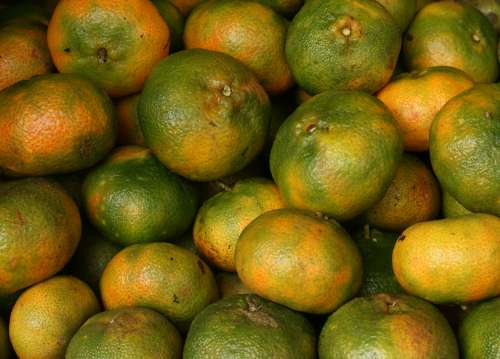The image depicts a large, haphazardly piled group of small citrus fruits, likely clementines or tangerines, viewed from above in a square-cropped frame. The majority of the fruits are predominantly green and unripe, with occasional hints of orange and yellow, indicating the early stages of ripening. Scattered among the fruits are a few orange-tinted ones, particularly visible in the upper left corner. Some of the fruits are oval-shaped, almost like flattened circles, and a few have small wooden stems. The overall arrangement is random, with the fruits lying on their sides or upside down. The chaotic pile obscures the surface they rest upon, leaving only subtle glimpses that suggest they might be in a box or on a display table.